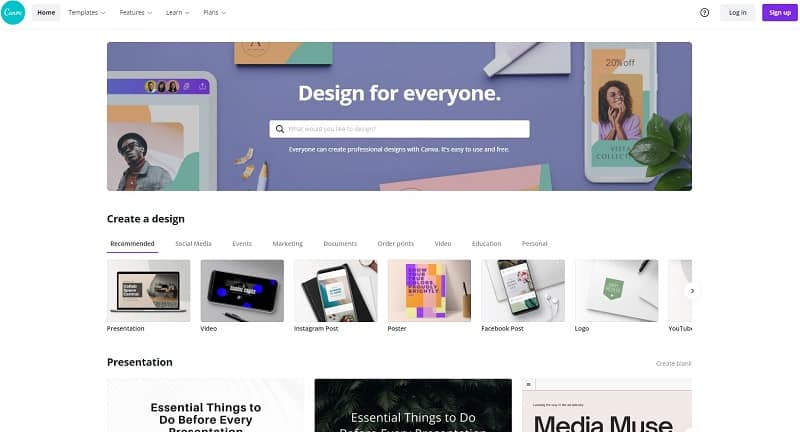The image is a screenshot of the Canva website, showcasing its user-friendly design and accessibility features. In the top left corner, a blue circle contains text in small white font that is difficult to discern. Adjacent to this, the primary navigation menu lists "Home," "Templates," "Features," "Learn," and "Plans," each with a dropdown arrow for additional options. To the right of these menu items, there is a circle with a question mark inside, followed by a "Login" button in black font on a white-light gray background. Next to it, a "Sign Up" button is displayed in a purple box with white font.

Below the navigation bar, a prominent headline reads, "Design for Everyone," in white font set against a blue-purple-gray background. A large white search bar underneath highlights the ease of using Canva with the text, "Everyone can create professional designs with Canva. Get Canva. It's easy to use and free." The interface also features visuals of a phone, an iPad/tablet, and other devices, indicating compatibility across multiple platforms. Menu categories such as "Create a Design," "Recommended," "Social Media," "Events," "Marketing," "Documents," "Order Prints," "Video," "Education," and "Personal" are listed prominently, each with accompanying icons. The diversity of devices depicted—including laptops and phones—underlines Canva's versatility for various design needs.